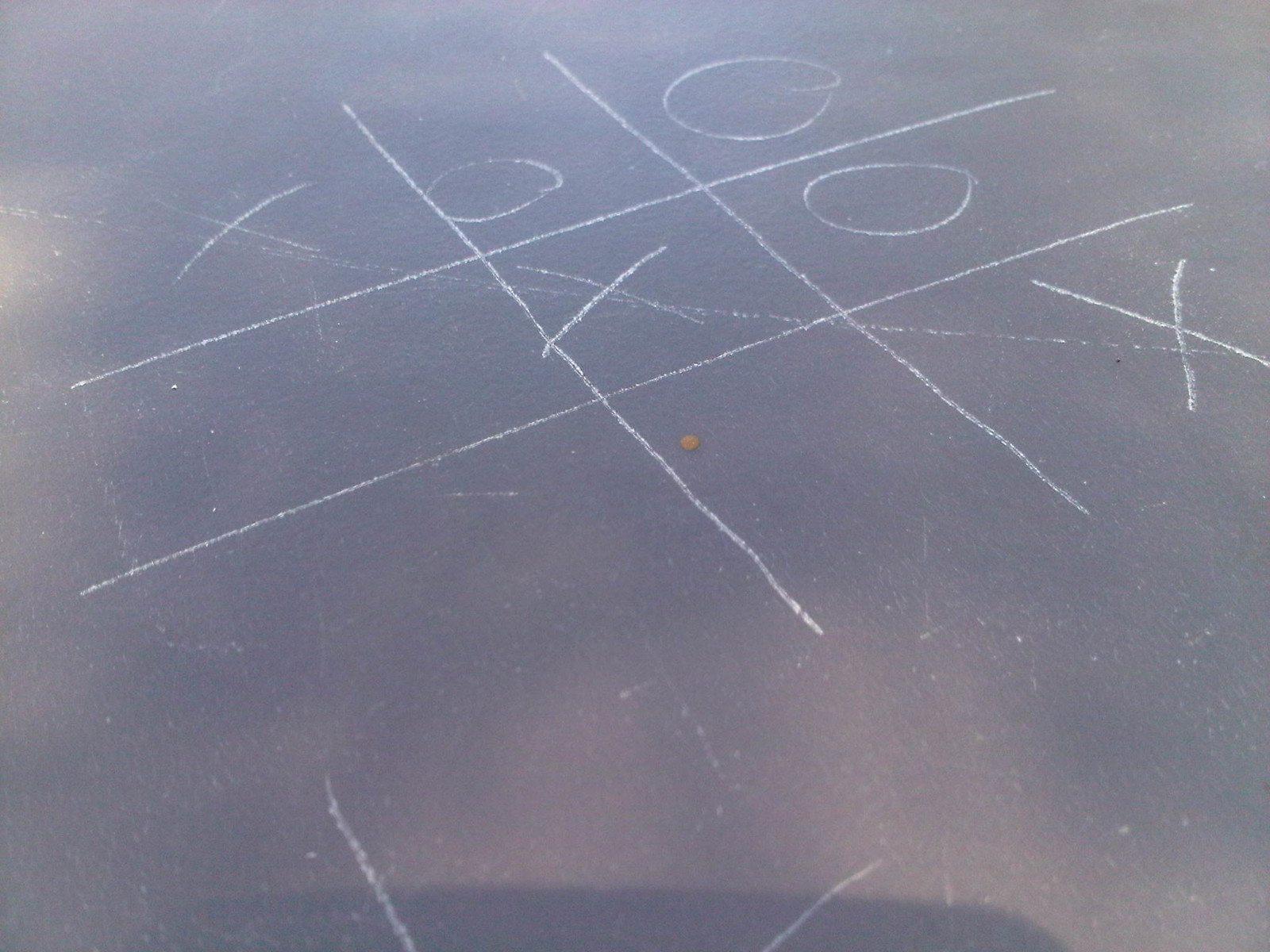The image shows a detailed chalk drawing of a Tic-Tac-Toe game on an asphalt surface. The board consists of crisscrossing vertical and horizontal lines forming nine distinct squares. In this game, one player has drawn three consecutive X's — one at the top left, one in the center, and one at the bottom right — successfully forming a winning diagonal line. A chalk line is drawn through these three X's to indicate the victory. The opposing player has placed O's in three of the remaining squares. The clear shadows at the very bottom center of the image add depth, but otherwise, the focus remains on the cleanly drawn Tic-Tac-Toe game, highlighting the winning X's.